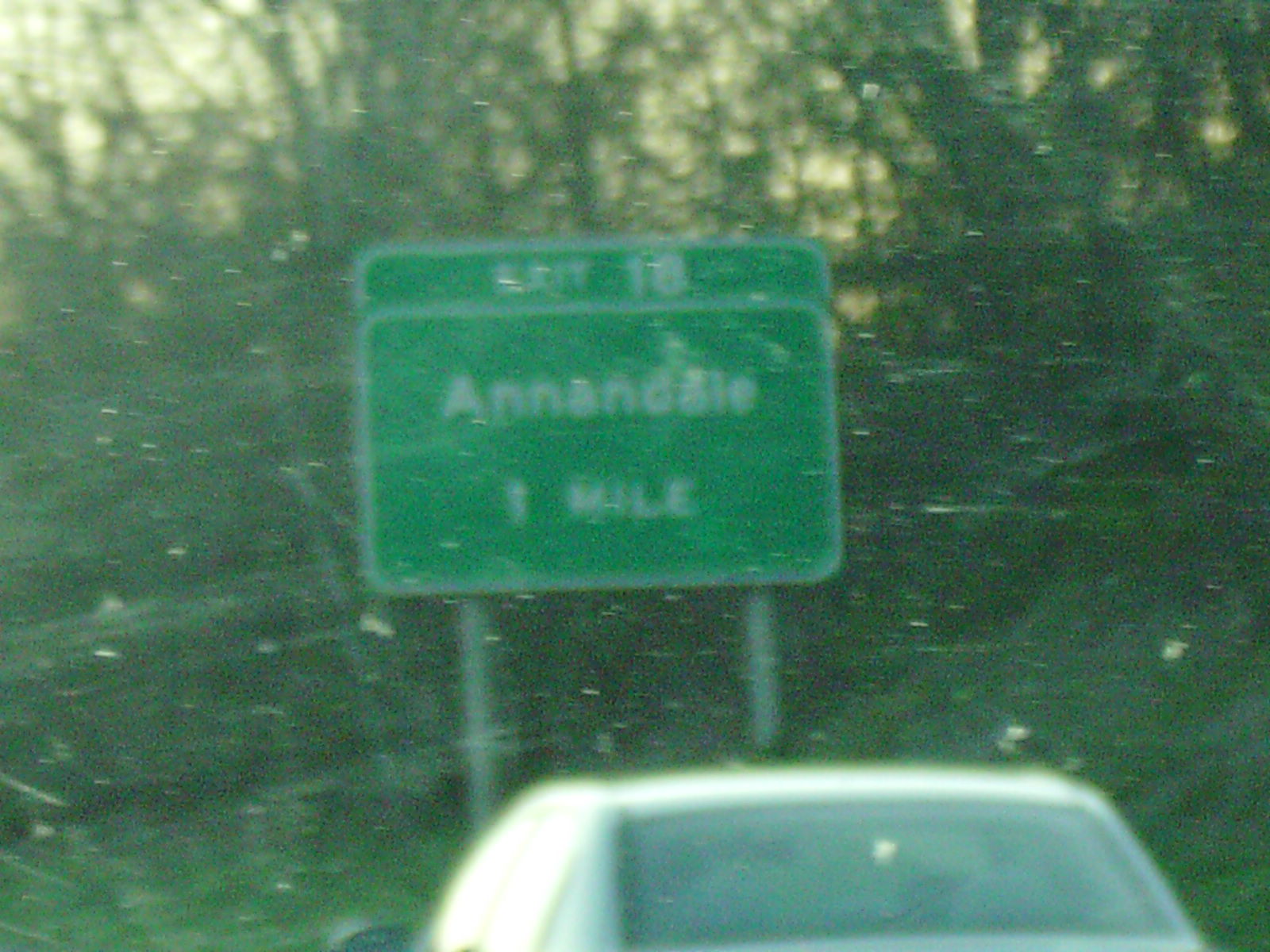This photograph captures a slightly distorted and blurry image of a green, rectangular road sign, adorned with tiny white specks that give it the illusion of being in the midst of a snowstorm—likely a result of the image's quality rather than actual snow. The sign prominently displays "Anna Dale" in white font, indicating a distance of one mile, with "Exit 18" written above. Beyond the sign, a dense wooded area with an intricate tapestry of trees and branches forms the background. At the very bottom of the image, the roof of a gray car is visible, suggesting movement alongside the sign, adding a dynamic element to the scene.